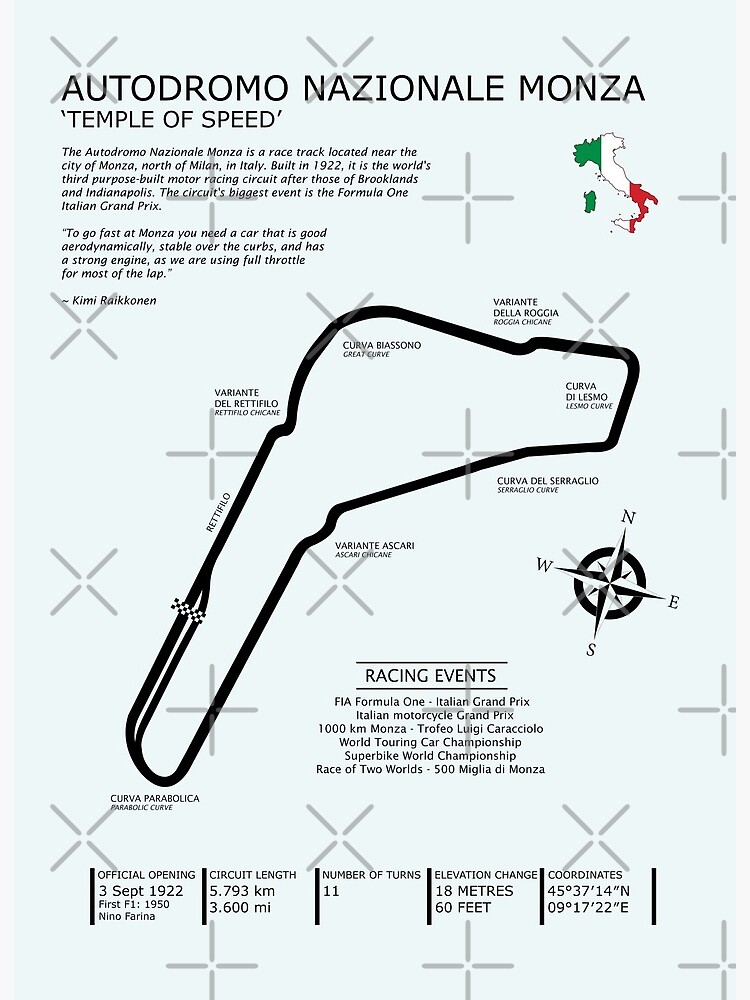The poster is an informative display about the Autodromo Nazionale Monza, prominently featuring the title "Temple of Speed" at the top in both Italian colors and the shape of Italy in the upper right corner. A detailed map of the iconic racetrack, which is located near the city of Monza, north of Milan, Italy, is at the center. Constructed in 1922, this historic circuit is celebrated as the world’s third purpose-built auto racing track. The map indicates the racetrack's L-shape and is surrounded by comprehensive data: its opening date, total circuit length, number of turns, elevation changes, and geographical coordinates. Additional elements include a compass and references to recent and significant racing events that take place here, accompanied by the flag colors of Italy—green, white, and red—enhancing the overall design.